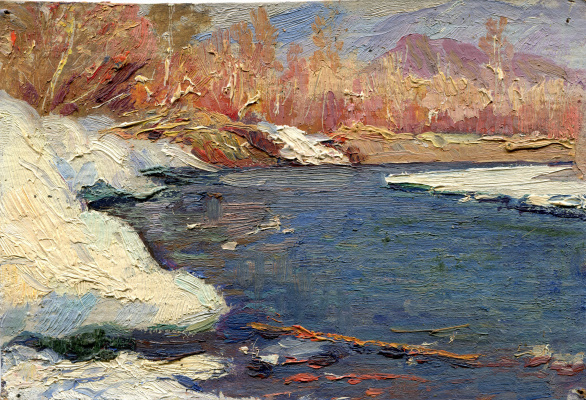The painting is an impressionistic depiction of a winter landscape, likely created using pastels or acrylics. The central focus is a river or creek with blue water, flowing toward the viewer, surrounded by snowy banks. The right bank is flat, while the left is more sloped and hilly, both covered in white snow and scattered with dead leaves and straw painted in orange and brown tones. Stylized, barren trees with light brown bark line the backdrop, extending into a wooded area. In the far background, a purple mountain range rises under a blue sky with hints of clouds. Accentuated brushstrokes and textured surface details exemplify the artist's technique, capturing a cold, serene winter scene devoid of green foliage.